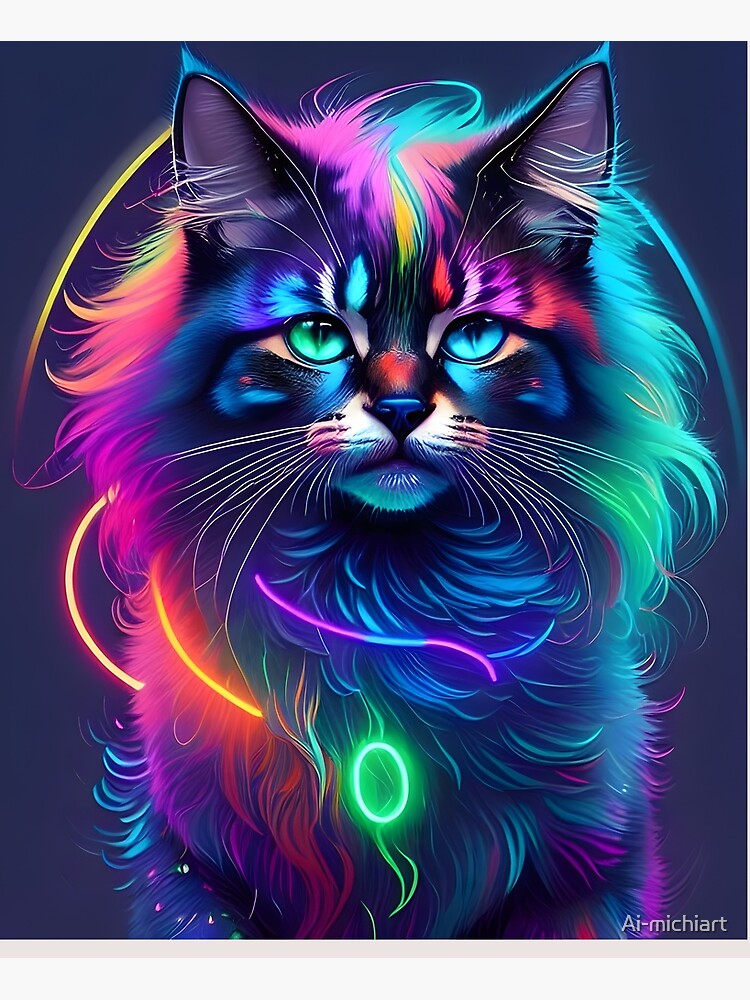The digitally created poster is a vibrant and futuristic depiction of a cat, marked by its neon and multicolored fur. Set against a black background with a faded purple hue, the image is infused with luminous colors that range from light blue and neon blue to vivid pinks, greens, reds, and yellows. The cat, adorned with intricate stripes and swirling patterns in hues of teal, orange, yellow, red, and purple, features bright blue eyes and rainbow-colored eyebrows. Its long mane and fur are highlighted, giving it a majestic appearance. The cat wears a collar, featuring a brightly lit green circular tag or possibly the letter "O." Bright white whiskers add to its striking and futuristic look. The bottom right corner bears the logo "AI-Michi Art," indicating its creation by artificial intelligence. The cat's intense gaze is directed straight at the viewer, adding to the captivating and otherworldly aesthetic of the illustration.